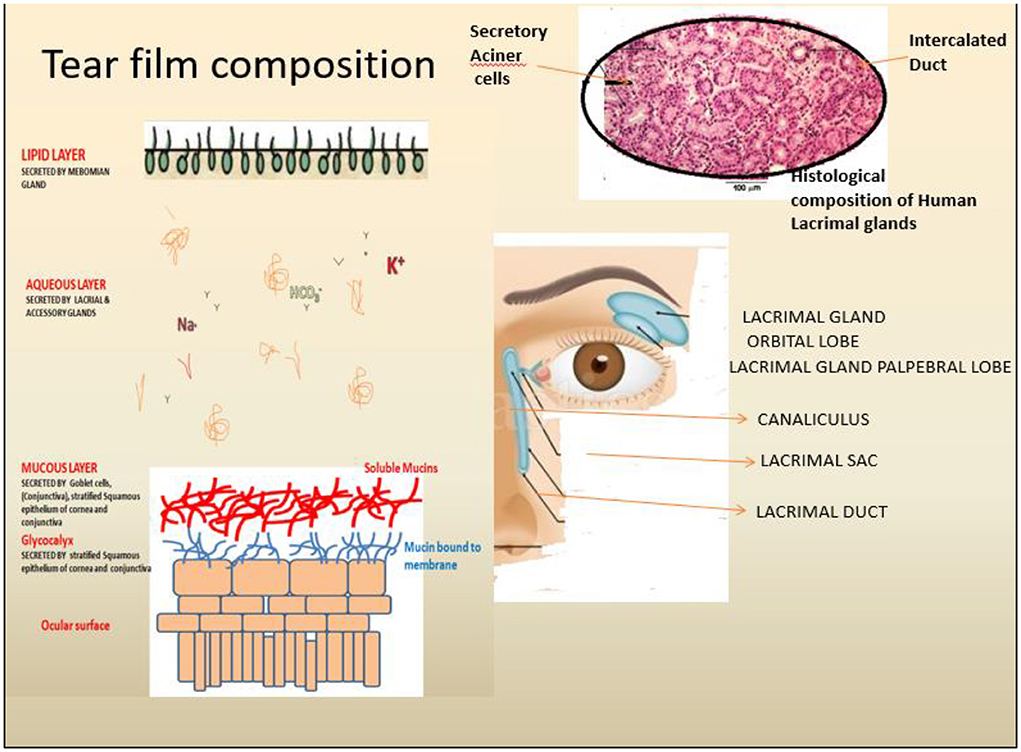This rectangular infographic, displayed in a landscape layout, meticulously details the composition and anatomy of the tear film. The overall background is a tan or cream color. The top of the infographic, bearing no border, is twice as long as the bordered left, right, and bottom sides that are lined with a thin black border.

Prominently positioned at the top left corner in black text is the title "Tear Film Composition." Adjacent to this, the term "Secretory Acinar Cells" is paired with an illustration of an oval containing various red cells. Below this, in the upper left section, three vertically aligned drawings in shades of green, cream, red, and blue, accompanied by black and red text, further describe the tear film's layers and compounds.

The right side of the infographic contains a more detailed anatomical section. Featured is a histology diagram of human lacrimal glands, with cells stained in pink, and an eyeball drawing complete with an eyebrow and surrounding ducts. These ducts are annotated with arrows leading to black text labels such as "Lacrimal Gland" and "Canaliculi," detailing each part's role in tear production and drainage. The bottom section of the infographic talks about the aqueous layer, including ions like potassium and sodium, and the mucus layer associated with the ocular surface, thus completing the comprehensive overview of the tear film composition and anatomy.